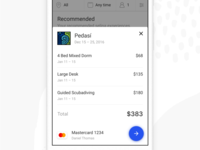The image is a highly detailed, edited screenshot of a purchase screen from the App Store. At the top of the screenshot, the word "App Store" is prominently displayed in the background. Below this, on the left side, the word "Recommended" appears in bold black letters, though still small in size. 

Beneath that, there is a white pop-up box featuring purchase options. In the top right corner of the pop-up, there is a small 'X' icon. On the left side of the pop-up, a game thumbnail is visible. To the right of the thumbnail, the game's name is displayed. 

The pop-up contains three items listed with their respective prices on the right side. At the bottom of the list, the word "Total" appears on the left side, with the cumulative price of all items—$383—displayed on the right. Additionally, the bottom left corner of the pop-up shows the user's MasterCard information, which has been automatically applied for the purchase. On the bottom right, there is a blue circle with a right-pointing arrow indicating the option to complete the purchase. 

Overall, the image depicts a user in the process of buying game add-ons, totaling $383.